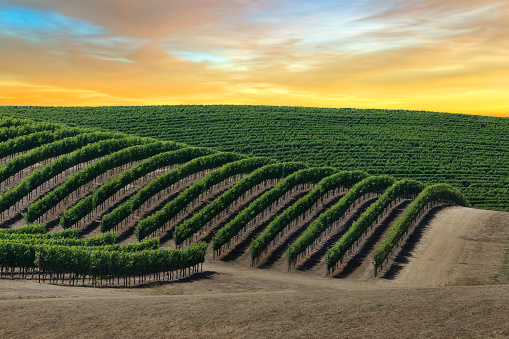The image showcases a picturesque vineyard sprawling across gently rolling hills, with meticulously aligned rows of lush green grape vines extending as far as the eye can see. The bare, earthy brown dirt between the rows accentuates the neatness of the plantation, creating a striking contrast. The setting sun casts a golden hue across the horizon, blending with the scattered clouds in the sky to paint a vibrant gradient of colors ranging from deep gray to rich gold, and deep blue to orange. The vast and idyllic landscape captures both the grandeur of the vineyard and the serene beauty of a tranquil evening, emphasizing the harmony between the orderly rows of grape vines and the majestic natural backdrop.